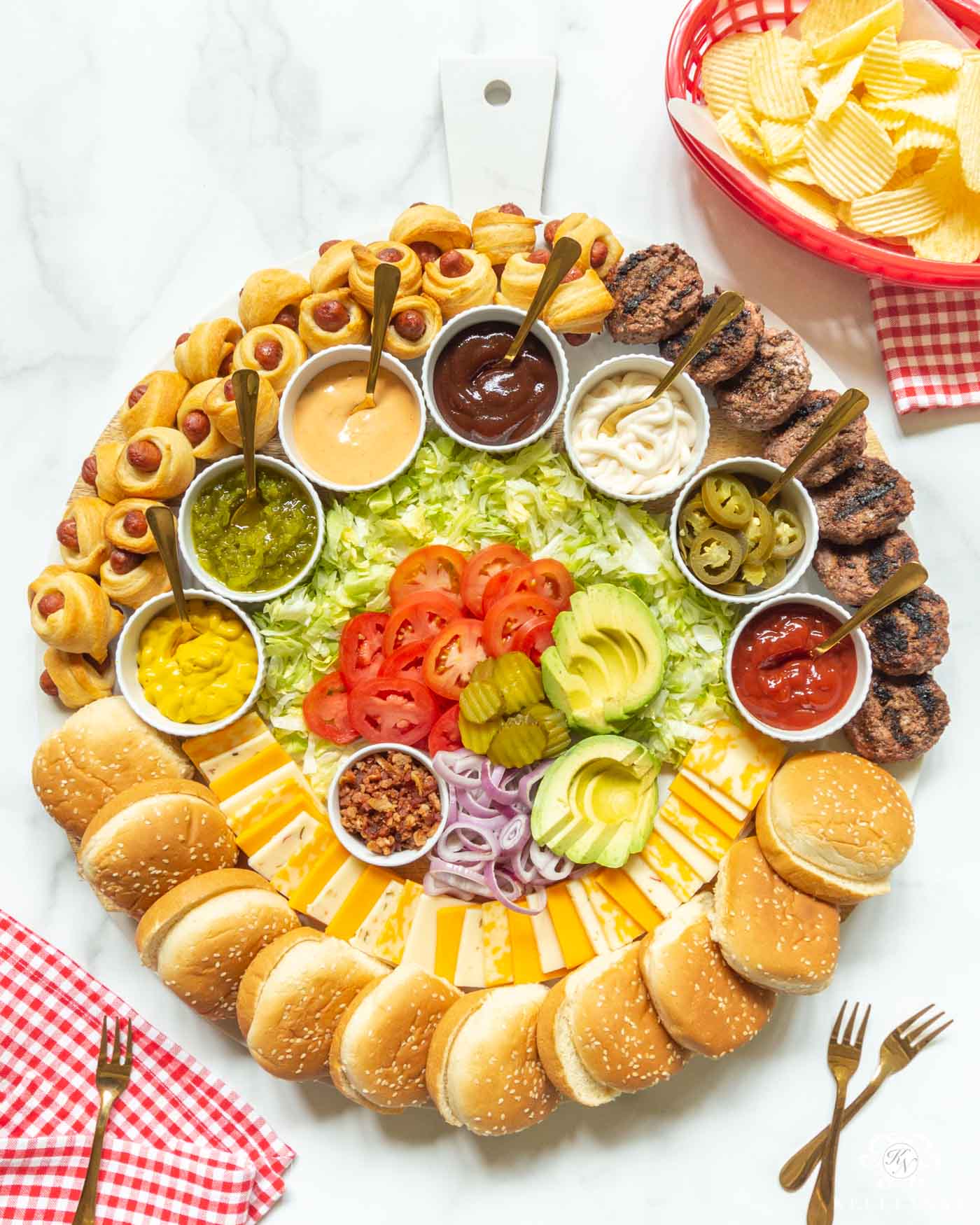The image depicts a large, gourmet round tray laden with an assortment of barbecue condiments and snacks, arranged meticulously. At the top left of the tray, small wieners wrapped in dough resembling baby pigs in blankets are nestled. Moving clockwise, there are mini hamburgers for sliders, and at the bottom third of the platter, small, round slider buns with sesame seeds. Surrounding the perimeter are small, white cups containing various condiments like mustard, relish, a yellow sauce, BBQ sauce, mayonnaise, hot peppers, and ketchup. 

In the center of the tray, on a bed of shredded lettuce, are arranged slices of tomatoes, avocados, pickles, purple onions, and bacon bits in a white cup, along with cubes of different cheese varieties such as cheddar, Colby, and pepper jack. Additionally, there is a red mesh container filled with ruffled chips, lined with a red and white checkered napkin, situated at the upper right corner of the picture. The lower left corner features another checkered napkin partially opened with a gold fork on it, and in the lower right corner, two gold forks are crisscrossed. The ensemble gives a gourmet and inviting feel, perfect for a barbecue feast.